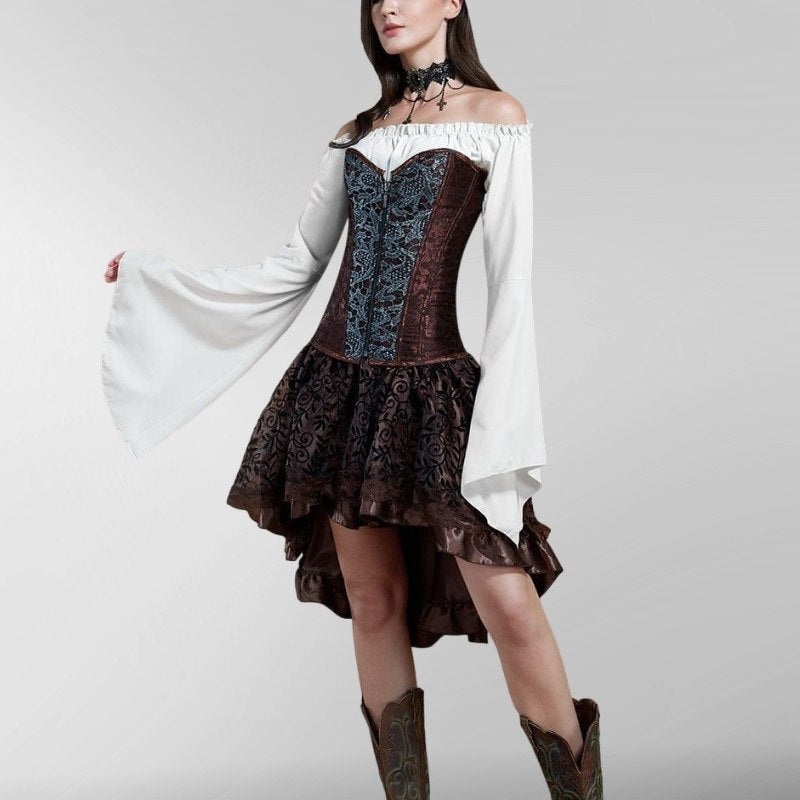The photograph portrays a young woman, only visible from the nose down to her ankles, standing against a gray backdrop. She is dressed in a striking Western-inspired ensemble, featuring a strapless dress with billowing white sleeves that extend artistically to cover her hands. The dress, a deep mauve or dark purple hue accentuated with intricate gray scroll designs, has a unique asymmetrical skirt—shorter in the front and longer in the back—embellished with a floral or plant pattern. The bodice, resembling a peasant style with a front zipper, is complemented by the dramatically large sleeves. She accessorizes with a choker adorned by a Christian cross along with other hidden adornments, and she dons high, brown leather cowboy boots that reach halfway up her calves, partially covering her thighs. The woman, leaning slightly to the side with one hand raised and the other relaxed by her side, sports long, dark brown hair and wears lipstick, adding to her elegant, yet rustic charm.